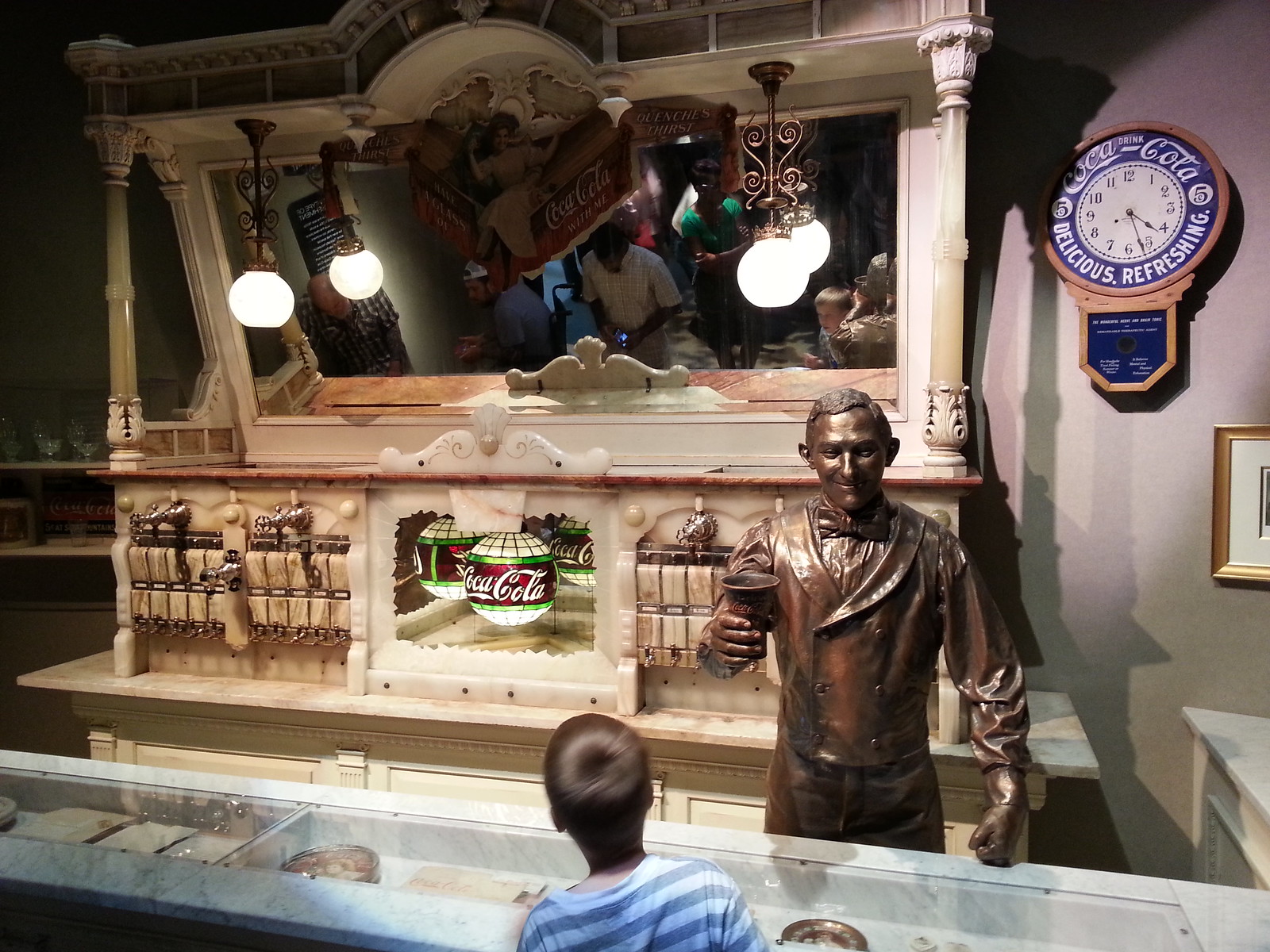The image is a surreal, colored photograph that seems as if it might have been created by AI. It features a small child positioned at the bottom edge, seen from behind, and wearing a stripy blue and lighter blue top. The child is standing before a glass display counter containing some indistinct, metallic objects. 

Central to the image is a bronze statue of a gentleman, resembling a 19th-century figure in a button-over jacket, possibly a soda jerk. The statue stands as though about to serve the child a drink. To the statue's right is a clock on the wall, which intriguingly has a blue edge and white face. The clock, likely a Coca-Cola one, carries the text "Delicious Refreshing" in white around its edge. 

Behind the statue, there’s a large cabinet with a slanted mirror, reflecting two white globe lights adorned with green and red labels, possibly advertising Coca-Cola. The area also includes variously positioned grey bottles or rectangular items. 

To the right, part of a picture in a gold frame is visible, as well as what appears to be a white table in the bottom corner. The left side of the image includes some shelving in a shadowed area. Reflected within the large mirror is a partial view of other individuals, adding to the nostalgic recreation of an old soda fountain.